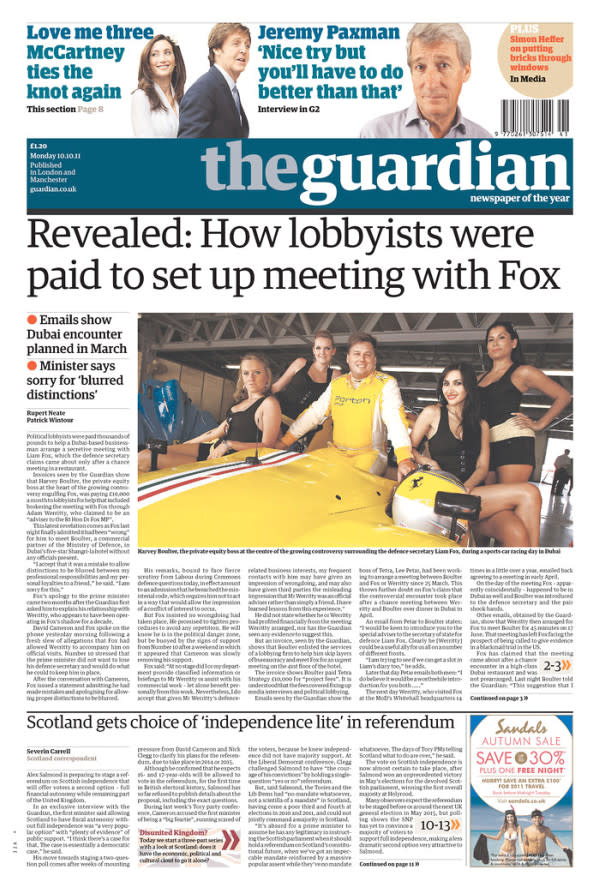The image is a screenshot of a newspaper page from The Guardian, identifiable by its distinctive blue header. The title "The Guardian" is positioned on the far right side of the header, with "the" in gray font and "Guardian" in white, all in lowercase. In the upper right-hand corner, there's a barcode. Above the main title, there is a photograph of a white man with gray hair, wearing a light gray shirt.

Next to this, the headline reads in blue font: "Jeremy Paxman: Nice try, but you'll have to do better than that." On the left side of this section, there is another headline stating, "Love Me 3: McCartney ties the knot again," accompanied by a photo of Paul McCartney and his new bride, who has long brown hair and is wearing a white shirt.

The main headline below The Guardian's name says, "Revealed: How lobbyists were paid to set up meetings with Fox." Beneath this headline is a photograph featuring several white women in black bathing suits.